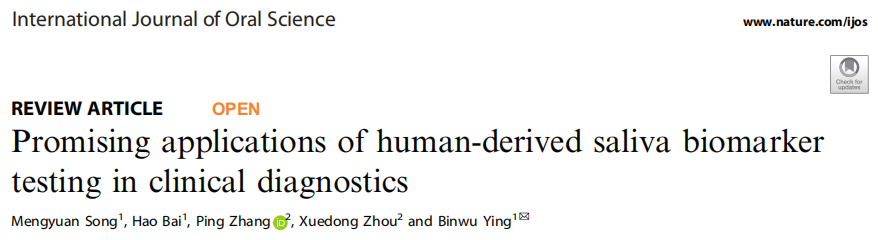The image is a screenshot of a headline from a scholarly website or an article from an online nature journal. The background is white, with text in a dark black or gray for clear readability. 

On the top left, it prominently displays "International Journal of Oral Science," indicating the publication's name. Correspondingly, on the top right, a URL is provided: www.nature.com/IJOS. Adjacent to this URL is a small gray box with the text "check for updates" in faint white letters, making it somewhat difficult to read. 

Additionally, there is a symbol featuring a circle with a flag inside, the significance of which is unclear. The headline of the featured article is crafted in bold and informative style, labeled as a "Preview | Review Article." 

An "Open" button in orange is positioned next to the title, inviting readers to access the full article. The headline declares, "Promising Applications of Human-Derived Saliva Biomarker Testing in Clinical Diagnostics," hinting at the article's scientific focus and potential impact.

Underneath the title, the authors' names and their respective affiliations are listed: Min Wang Song (#1), Hao Bai (#1), Ping Zhang (#2), Zui Dong Zhao (#2), and Bin Wing Ying (#1), presumably indicating their contributions and institutional associations.